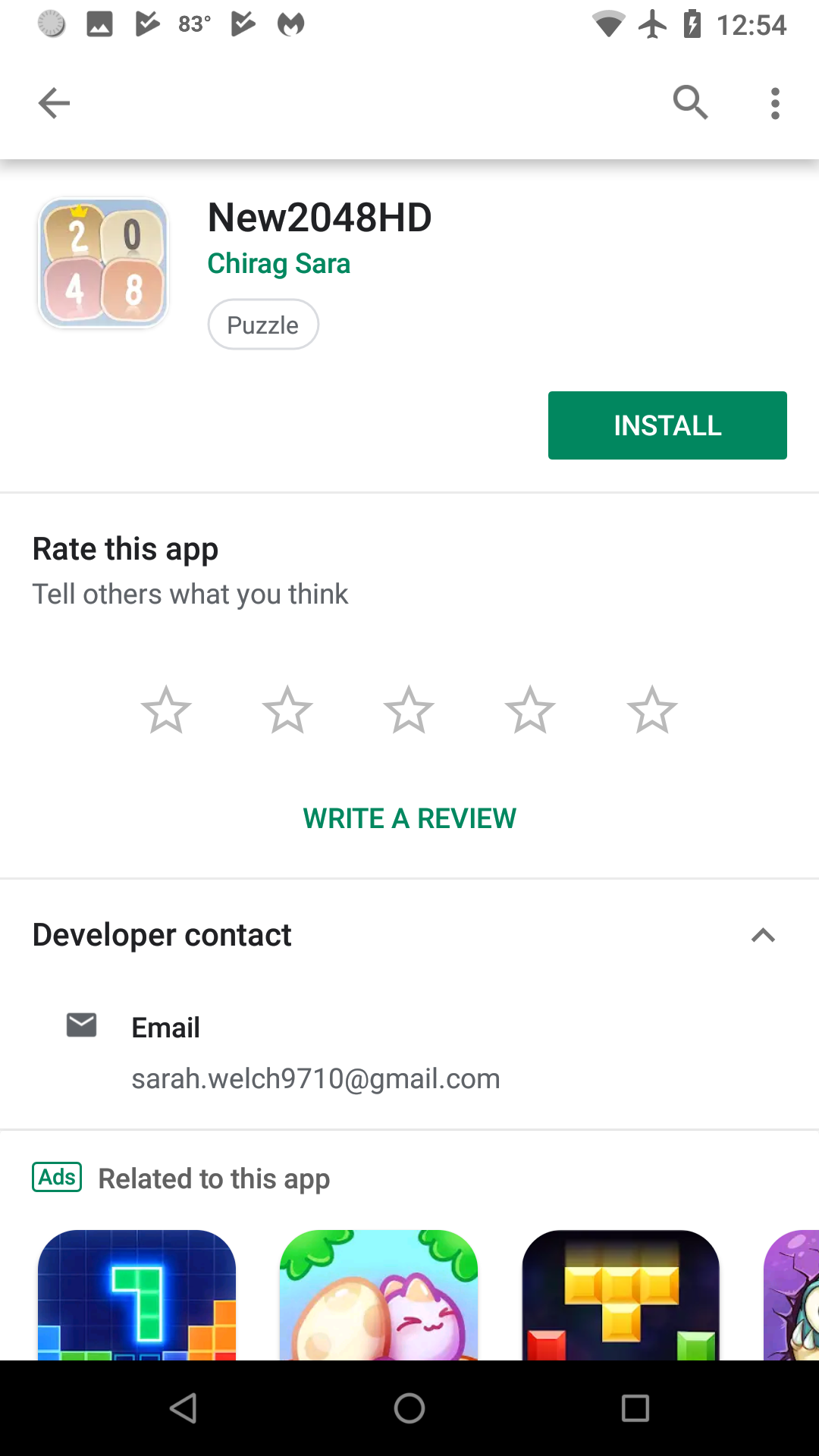This is a detailed cell phone screenshot depicting an app information screen. At the very top, there is a standard line of status icons in gray, indicating elements like signal strength, Wi-Fi, and notifications. The time and battery percentage are prominently displayed on the right side. Below this line, there is a gray arrow pointing left on the left side, and on the right side, a gray magnifying glass icon is adjacent to a vertical ellipsis (three dots).

Further down, a gray horizontal divider line spans across the width of the screen. In the upper left-hand corner beneath this line, there is a distinct square icon featuring a 2x2 grid. The grid contains four smaller boxes: the top left box has a brown background with the white number "2," the top right has a tan background with a black "0," and both bottom boxes have brown backgrounds—with the left showing a white "4" and the right a white "8."

To the right of this icon, bolded black text reads "2048HD." Directly below this, in green text, it states "C-H-I-R-A-G Sarah." An oval outlined in gray appears below this, containing the word "Puzzle" in gray text.

A few lines down and aligned on the right side, a green rectangle with white text reads "Install." Another gray horizontal line follows this, leading to a section titled "Rate this app" in bolded black text. Below it, in gray text, the prompt "Tell others what you think" encourages feedback. 

Centered a few lines below this, the gray outline of five stars invites users to rate the app. Beneath the stars, the phrase "WRITE A REVIEW" is bolded and in all caps green. The section "Developer contact" follows, captioned in bolded black text. Accompanied by a letter icon, the word "Email" appears in bold black, with the developer's email address listed directly underneath.